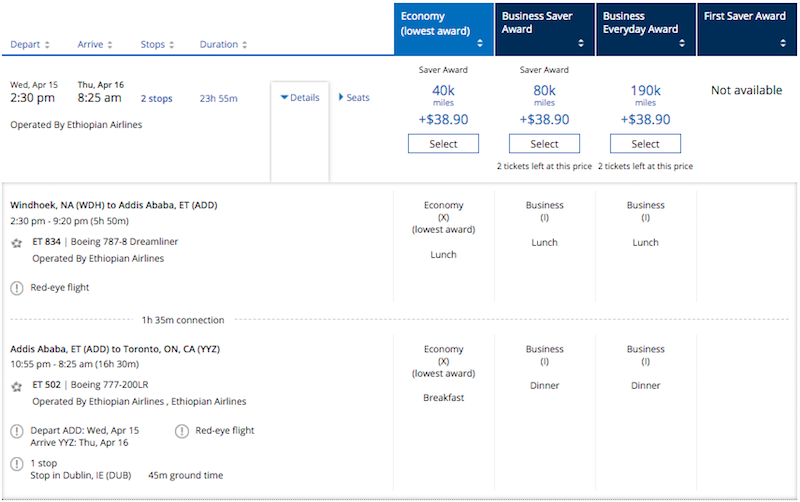**Detailed Caption:**

This image shows an itinerary for a multi-leg international flight. In the top-left corner, flight details are laid out, including "Depart," "Arrive," "Stops," and "Duration," along with various award types such as "Economy," "Lowest Award," "Business Saver Award," "Business Everyday Award," and "First Saver Award."

**Flight Information:**
- **First Leg:** 
  - **Departure:** Wednesday, April 15th at 2:30 PM
  - **Arrival:** Thursday, April 16th at 8:25 AM
  - **Operational Details:** Ethiopian Airlines with two stops over a duration of 23 hours and 55 minutes.
  - **Class Options and Prices:** 
    - First Saver Award: 40km + $38.90
    - Economy Saver Award: 80km + $38.90 (two tickets left at this price)
    - Business Saver Award: 80km + $38.90
    - Business Everyday Award: 190km + $38.90

- **Connecting Flights:**
  1. **Flight from Windhoek (WDH) to Addis Ababa (ADD):**
     - **Departure:** 2:30 PM 
     - **Arrival:** 9:20 PM
     - **Duration:** 5 hours and 50 minutes
     - **Flight Number:** ET834
     - **Aircraft:** Boeing 787 Dreamliner, operated by Ethiopian Airlines
     - **Class Amenities:** Economy, Business 1, and Business 2 classes are available with lunch served
     - **Flight Type:** Red-eye flight
     - **Connection Time:** 1 hour and 35 minutes

  2. **Flight from Addis Ababa (ADD) to Toronto (YYZ):**
     - **Departure:** 10:55 PM 
     - **Arrival:** 8:25 AM (April 16th)
     - **Duration:** 16 hours and 30 minutes
     - **Flight Number:** ET502
     - **Aircraft:** Boeing 777-200LR, operated by Ethiopian Airlines
     - **Class Amenities:** Economy, Business 1, and Business 2 classes with breakfast and dinner served
     - **Flight Type:** Red-eye flight with one stop

The detailed flight details provide insights into the comprehensive travel plan, ticket options, prices, and amenities, ensuring the traveler is well-informed for their journey.